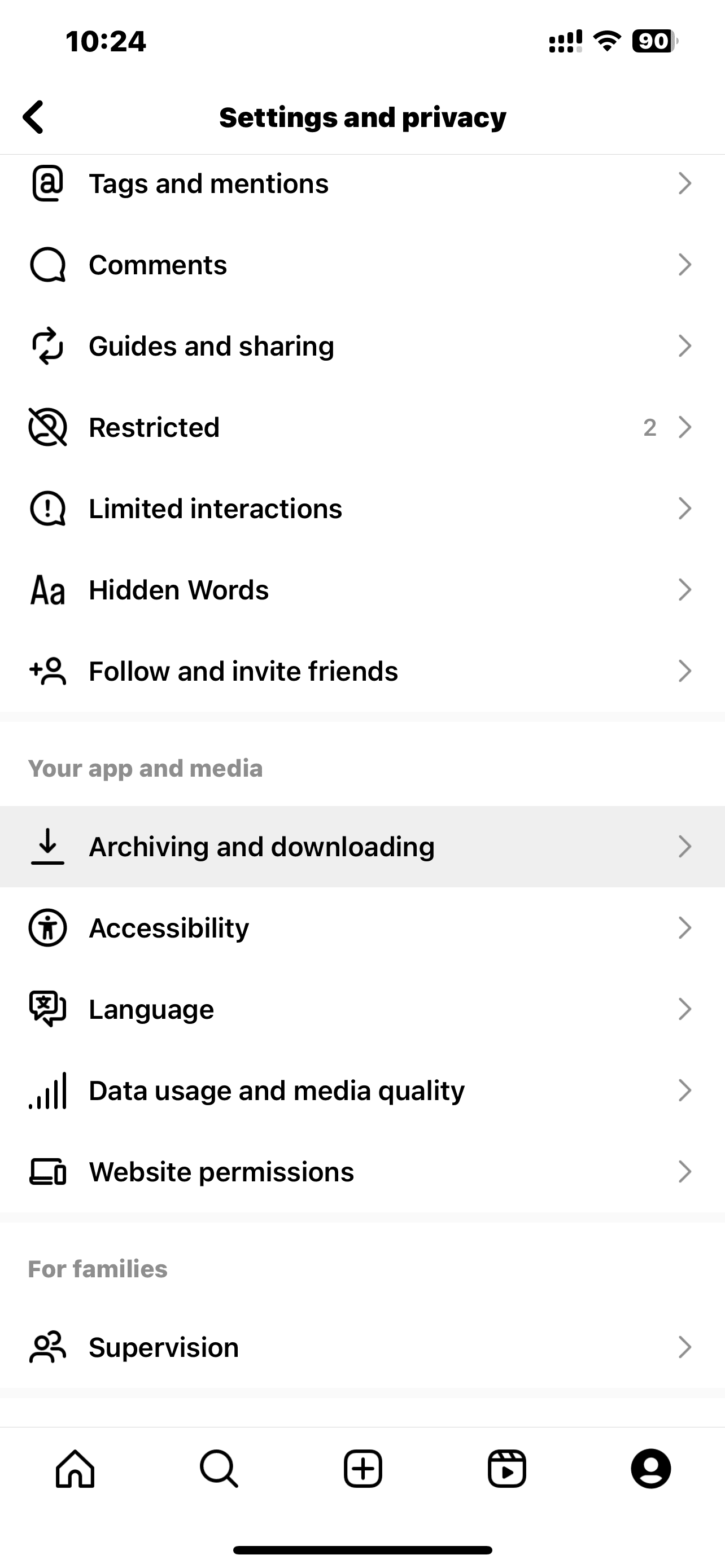The image depicts a cell phone screen displaying its current status and settings interface. At the top of the screen, the time is shown as 10:24, with the status indicators to the right: a signal strength bar displaying 4 bars, a Wi-Fi symbol indicating an active connection, and a battery icon showing 9% charge remaining. 

Below the status bar, the screen displays the 'Settings and Privacy' menu, emphasized in bold print. This main heading has been selected from a previous menu. The options listed under this heading include:

1. **Tags and Mentions** 
2. **Comments** 
3. **Guides and Sharing**
4. **Restricted** (noted with a number 2 beside it)
5. **Limited Interactions**
6. **Hidden Words**
7. **Follow and Invite Friends**

Each of these options features a small arrow (caret) symbol, indicating expandable submenus.

Further down, a subheading titled 'Your App and Media' encompasses a list of additional settings:
- Archiving and Downloading
- Accessibility
- Language
- Data Usage and Media Quality
- Website Permissions

Another section, labeled 'For Families,' contains a solitary option for 'Supervision.'

At the bottom of the screen, a navigation bar displays five icons typically found on many apps: a house symbol for the home screen, a magnifying glass (search), a plus sign (add content), a video icon, and an account symbol.